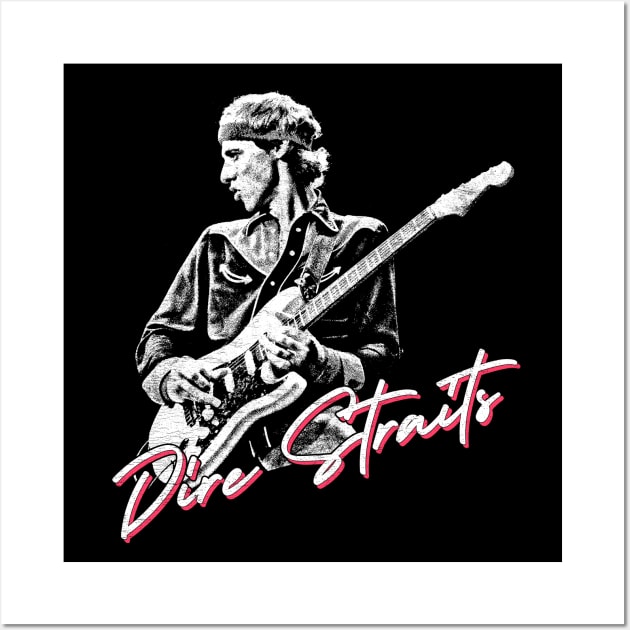This black-and-white graphic artwork from the 1980s features a detailed depiction of a guitarist. The image is framed by a white border, enclosing a central black square, within which the guitarist is rendered in white, creating a stark contrast. He is seen wearing a loose, casual, long-sleeve button-up shirt with the top two buttons undone, indicative of a relaxed style. A headband wraps around his head, adding to the quintessential 80s aesthetic. His facial features and the details of his shirt are clearly visible against the black background. The guitarist is holding an electric guitar, his right hand poised to strum while his left hand grips the neck. Beneath his image, the words "Dire Straits" are prominently displayed in white text with a pink-red shadow, creating a 3D effect that overlaps part of the guitarist's figure. The overall theme and elements of the artwork exude a strong 80s vibe.